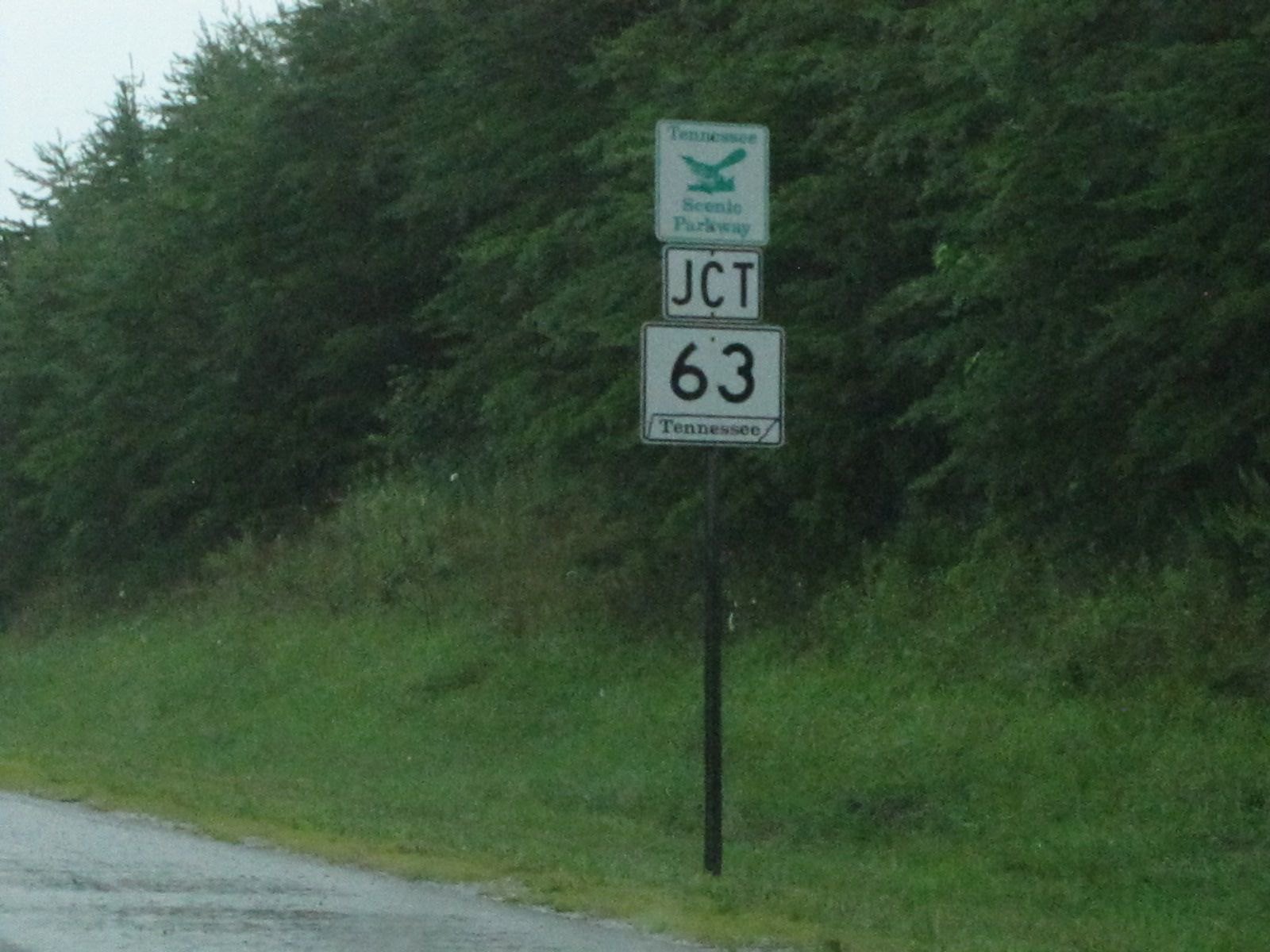This photograph captures a tranquil scene featuring a roadside area bordered by lush greenery. In the background, the top left corner reveals a slightly pixelated, bluish sky, creating an ambiguous time of day. The backdrop showcases an array of green trees and overgrown shrubbery, extending across most of the image. The foreground presents a gradual transition from high grass in the middle to shorter grass towards the bottom of the frame, where a cement or gravel road becomes visible on the left side.

Anchoring the center of the image is a black pole supporting three distinctive signs. The top sign, adorned in green, proclaims "Tennessee Scenic Parkway" alongside a depiction of an eagle. Directly beneath it, a rectangular sign displays "JCT" in bold black letters within a black border. The bottom square sign identifies "Tennessee" and "63" in black lettering against a light-gray background. This scene, likely indicative of a park or natural area, is bordered by a small ditch running alongside the road, emphasizing the connection between manmade infrastructure and nature.